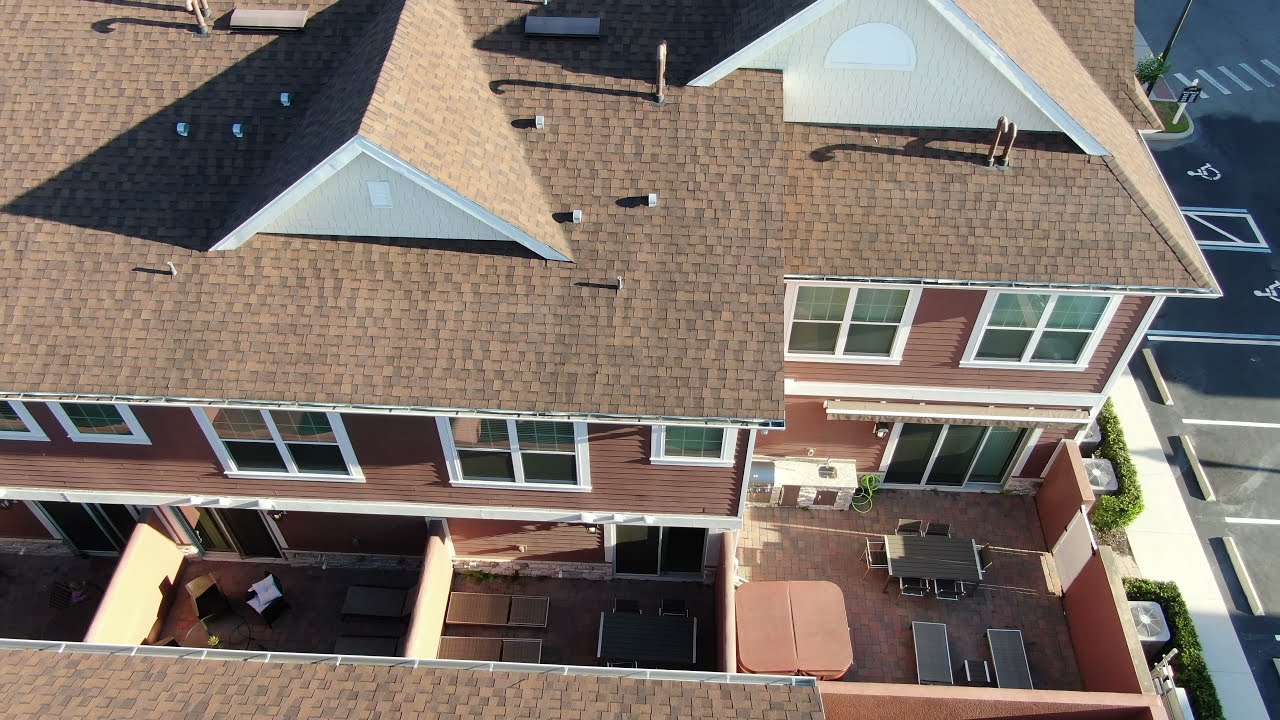This detailed aerial photograph captures the rear view of a multi-story apartment complex, taken from a drone-height of about 30 feet. The building, characterized by its red siding and large white windows, has a brown-tiled roof adorned with triangular white architectural features. To the right of the image, a parking lot is visible, complete with marked handicap spaces and crosswalk lines. The rear of the building reveals multiple small, concrete-paved backyards or patios for each unit, separated by dividers. These outdoor living spaces are furnished with tables and chairs, and one patio features a covered hot tub alongside a grilling section and a picnic table with six chairs. The main colors in the image include off-pink, brown, and white from the building and asphalt gray from the parking lot lines. No people, vehicles, or animals are present in the scene.